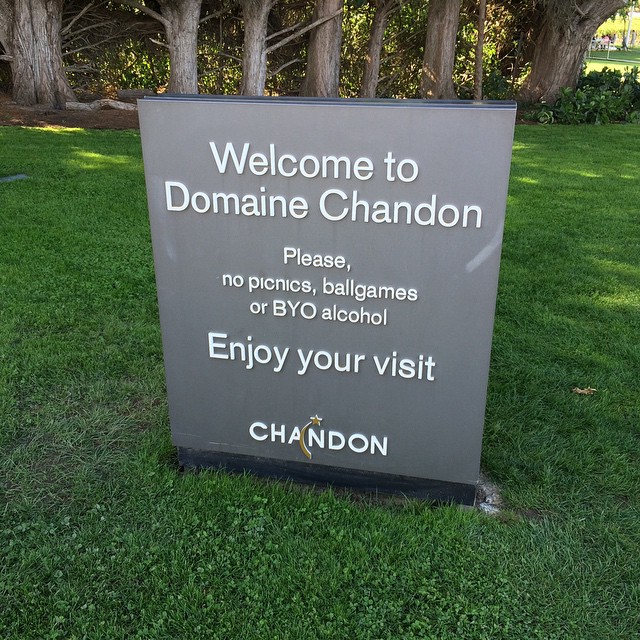The outdoor image captures the entrance to a park named Domaine Chandon. In the foreground, a gray rectangular sign with white text stands in a lush green lawn. The sign warmly welcomes visitors with the message: "Welcome to Domaine Chandon. Please, no picnics, ball games, or bring your own alcohol. Enjoy your visit." At the bottom of the sign, the name 'Chandon' appears, featuring a distinctive shooting star logo between the A and the N. In the background, old gray tree trunks stand in a row, with sunlight filtering through their branches, casting a serene glow on the greenery below.